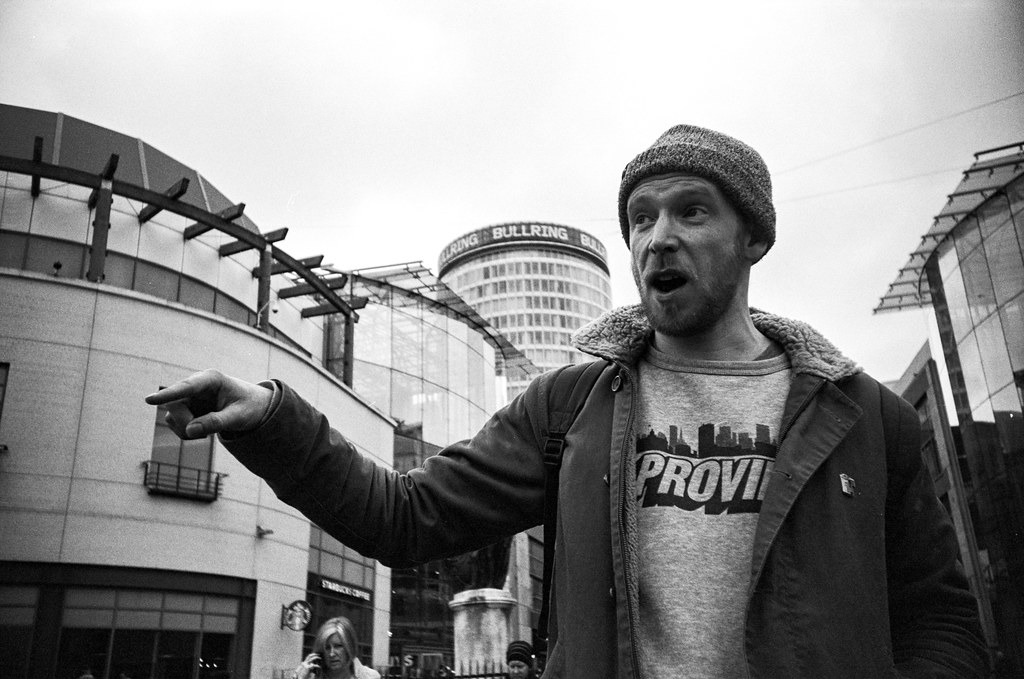This black and white photograph captures a close-up of a bearded man wearing a knit beanie and a heavy jacket with a fleece collar, accompanied by a sweatshirt underneath. An indistinct word, starting with "PROV," appears on his sweatshirt next to a skyline design. The man, who has his mouth slightly open and his right hand raised as if emphasizing a point, looks off to the side somewhat derisively. The backdrop reveals an overcast sky and various buildings that form what seems to be an outdoor shopping area. Prominent structures include a tall, circular building labeled "Bullring," a glass-walled building to the right, and further rounded buildings, with one bearing a Starbucks logo at the bottom. There are two women in the scene, one on her phone in the foreground and another walking in the distant background. The photo's perspective, from the man's waist up, suggests an intimate conversation or impassioned declaration in an urban setting.